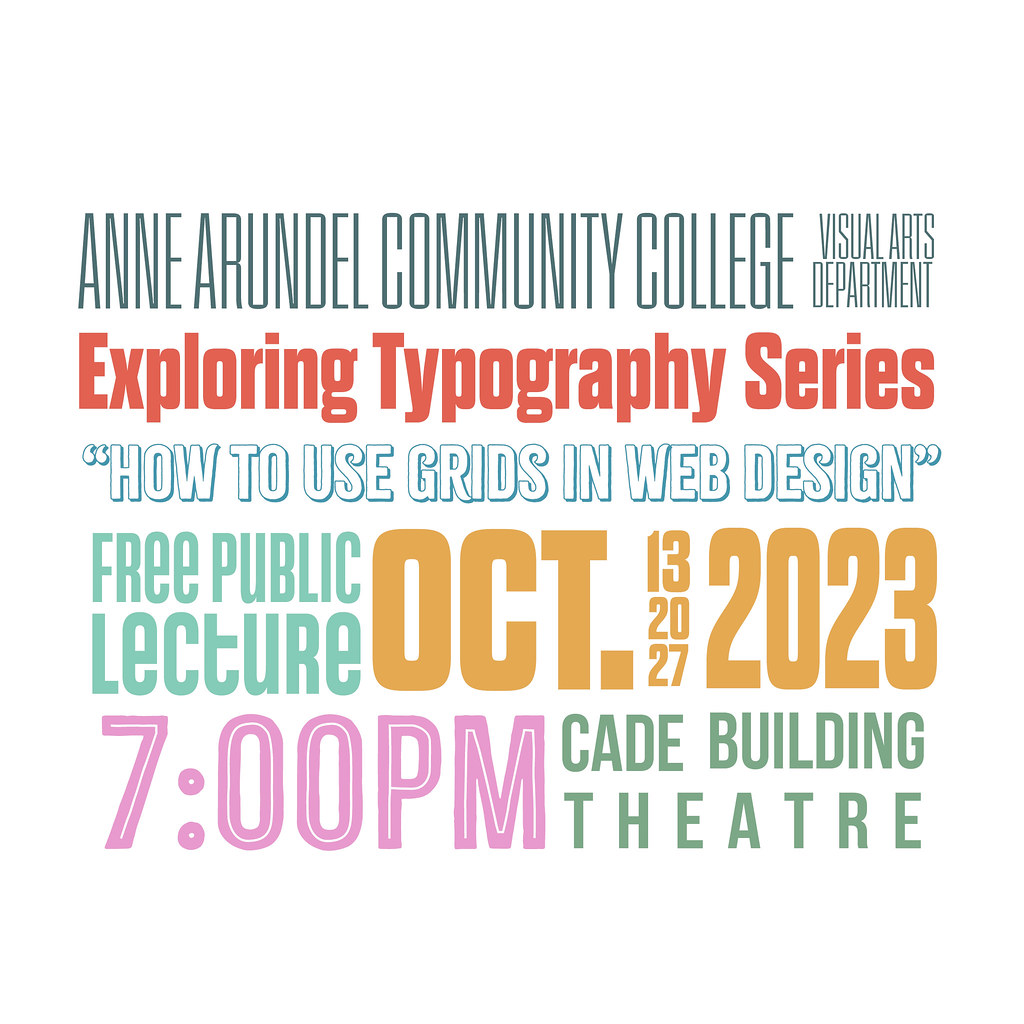The image is a promotional flyer featuring an array of text in various colors, fonts, and sizes on a white background. At the top, in thin, dark greenish-blue letters, it reads "Anne Arundel Community College." Adjacent to this, in a smaller but bold red font, it states "Visual Arts Department." Following this, in all capital letters, it notes "Exploring Typography Series" in a prominent red color. Below, in hollow blue letters with a white fill, the title "How to Use Grids in Web Design" is enclosed in quotes. Further down, the phrase "Free Public Lecture" appears in large bold green letters. Positioned to the right, in vivid yellow, it marks the dates "October 13, 20, 27, 2023." At the bottom left of the flyer, the time "7 p.m." is displayed in purple, while on the bottom right, the location "Cade Building Theater" is in a jade green font.